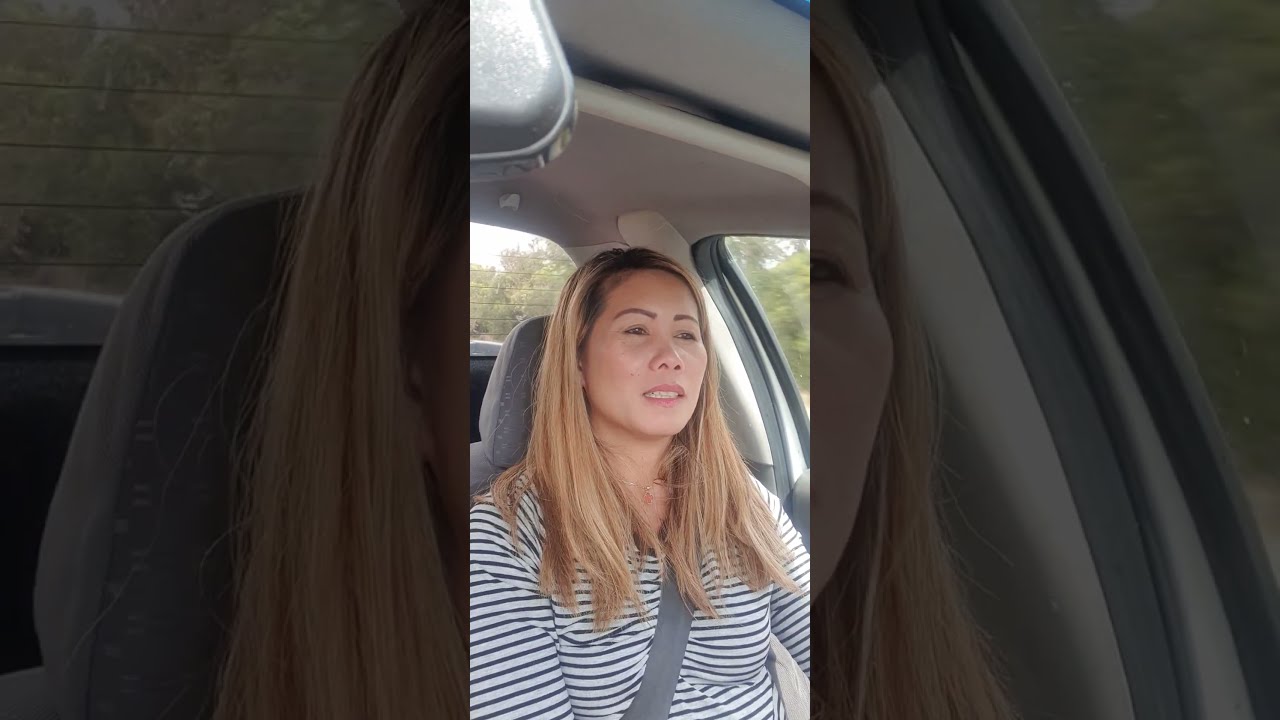The image appears to be a still from a cell phone video, potentially a TikTok, in portrait orientation. It features a woman of Asian descent with dyed dirty blonde hair, which shows black roots, seated in the driver’s seat of a car. She is wearing a black and white horizontally striped shirt and is secured with a seatbelt. The woman, whose skin tone is darker than white, is staring straight ahead, possibly addressing the camera, with her mouth partially open and teeth visible as if she’s talking. The car's interior has gray seats, and through the open driver’s window and the rear window with grid lines, the daylight sky appears mostly white with a hint of blue. The surrounding environment includes numerous green-leafed trees visible through the windows. The rearview mirror is also slightly visible near the edge of the frame.